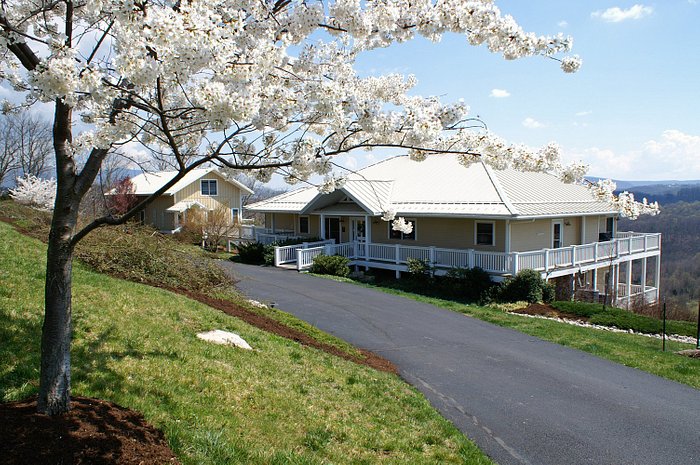In this picturesque daytime scene, a tranquil landscape unfolds under a light blue sky dotted with white clouds. A well-maintained road stretches from the bottom right and weaves its way to the middle left, eventually obscured by a grassy hillside adorned with bushes. Prominently positioned on the left side of the image, a small but fully grown tree boasts an array of delicate white blossoms, adding a touch of natural beauty. The foreground's grounds are pristine and free of flowers, further highlighting the tidy nature of the area. 

In the background, a standout feature is a large, multi-story house with a surrounding white patio deck. The house’s beige or light yellow walls contrast elegantly with its white roof. Despite the serene setting, there are no people or animals in sight, emphasizing the quiet and peaceful nature of the scene. The distant backdrop reveals expansive fields, additional trees, and rolling hills, completing the idyllic, scenic view.